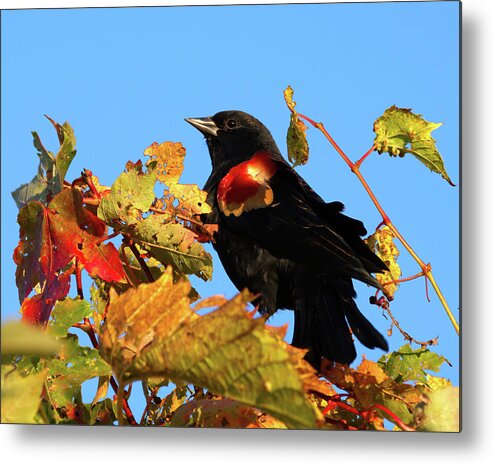This detailed image showcases a black bird perched atop a tree branch against the backdrop of a vividly bright blue sky. The bird, facing left and looking slightly upward, possesses a striking silvery gold beak and dark eyes. Its plumage is primarily black, with a distinct red patch where the wing begins, indicative of a red-winged blackbird. The leaves surrounding the bird are in the midst of autumn transformation, presenting a spectrum of colors: predominantly green at the base, transitioning to red, orange, and yellow at the tips. The leaves appear weathered and broken, some with holes suggesting insect activity or frost damage. Framing the image is a thin black border, reinforcing that the picture might be a photograph printed on canvas against a white wall.